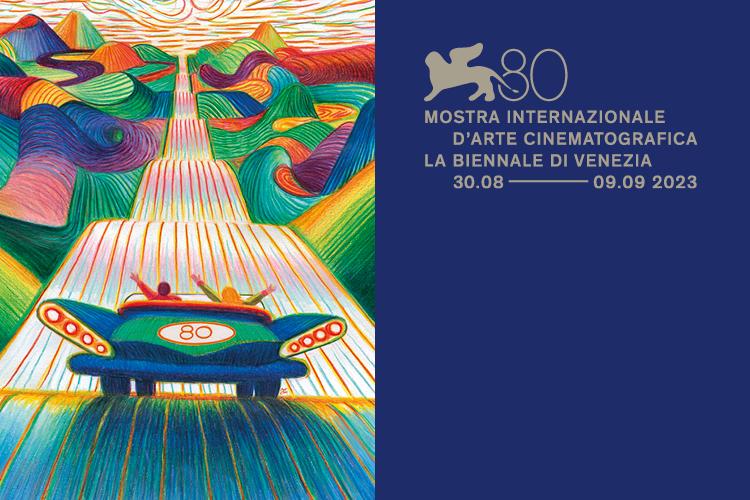This vibrant, rectangular image, with text on the right and an illustration on the left, appears to be an announcement. The left side features an eye-catching illustration of a classic green car, adorned with the number 80 in a white circle on its trunk. The car cruises down a dramatically hilly, iridescent road that dips and rises in vibrant, multicolored waves. Flanking the road are abstract, ribbon-like hills in blues, greens, and a spectrum of rainbow hues, creating a whimsical, kaleidoscopic landscape. Two passengers are visible in the car, both animatedly raising their arms: the person on the left, in a red shirt, extends their left arm, while the blond-haired person on the right has both arms lifted. The road, with its alternating red, yellow, and pink hues, stretches into the horizon, surrounded by swirling, colorful shapes. The right side of the image is a solid blue vertical box with white text, possibly an invitation in Spanish, accompanied by a small logo, highlighting the details of an event with dates and possibly the name "Mostra Internazionale d'Arte Cinematografica la Biennale di Venezia, 30.0A, 09.09-2023."